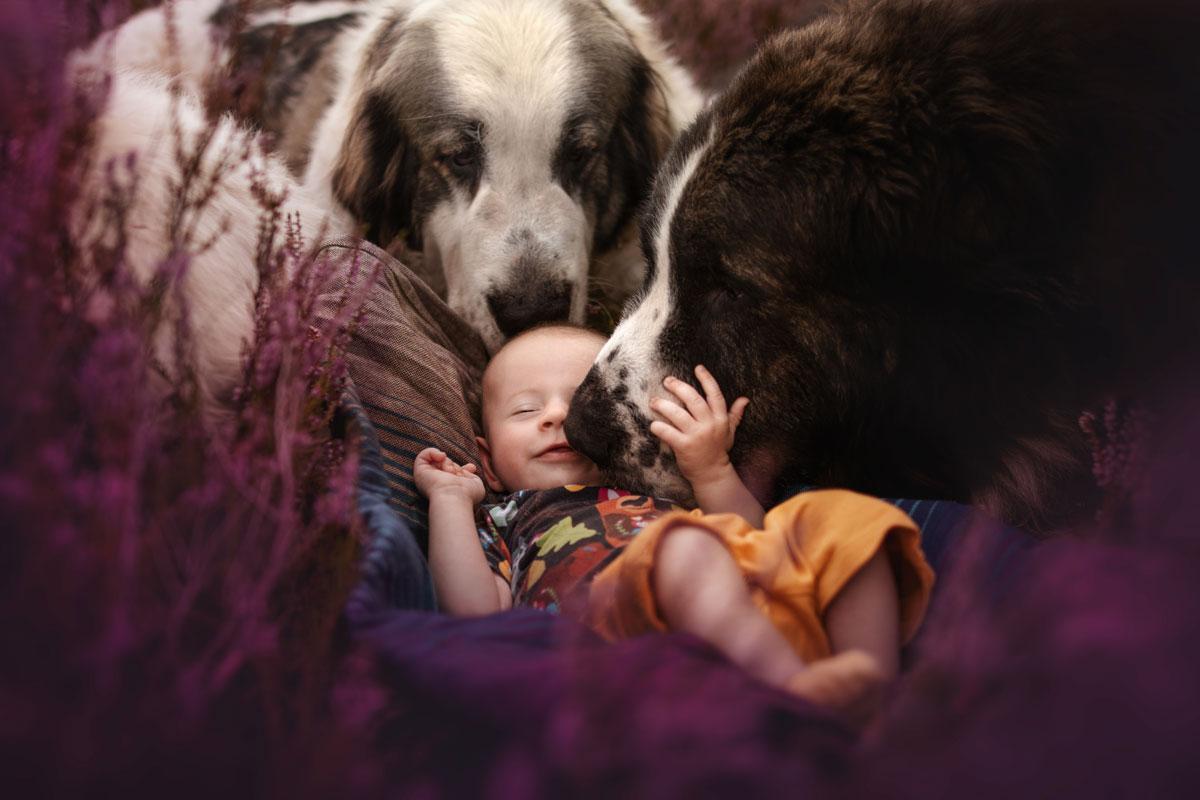The photograph captures a tender moment of a Caucasian baby, approximately four months old, reclining on a blue blanket with a background that includes a brown couch. The baby boy, dressed in orange pants and a multicolored, leafy-patterned shirt with a brown base, is smiling with his eyes closed. His partially bald head shows a bit of brown fuzz. Two large, affectionate dogs, resembling St. Bernards, are nuzzling close to him. The dog to the right, predominantly dark brown with a white stripe down its face, gently presses its nose against the baby's face, while the second dog, with a predominantly white coat and brown spots, lovingly nuzzles the top of the baby's head. The scene exudes warmth and contentment, emphasized by the baby’s hand resting on the dark brown dog’s face. In the foreground, purple flowers add a touch of color and softness to this heartfelt scene, capturing a sense of protective love and serene happiness.